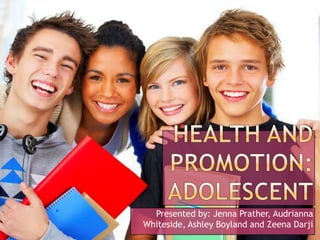The image is an advertisement with a nostalgic 90s vibe and a clean white background. It features four smiling students, likely aged 16 or 17, indicative of middle or high school. Arranged from left to right, there is a brunette boy with spiked hair wearing a gray sweatshirt patterned with blue, black, and white triangles. He carries three books in red, tan, and blue, and has headphones around his neck. Next is a dark-skinned girl with short hair and a white shirt. Standing beside her is a fair-skinned girl, possibly Hispanic, followed by another fair-skinned boy. The text overlaid on the image reads, "Health and Promotion Adolescent," in a plum-colored box, with a plum-colored rectangle below listing the presenters: Jenna Prather, Adriana Whiteside, Ashley Boyland, and Zena Darji. The teens’ joyful expressions and the well-coordinated visual elements suggest it could be a student project or promotional campaign.